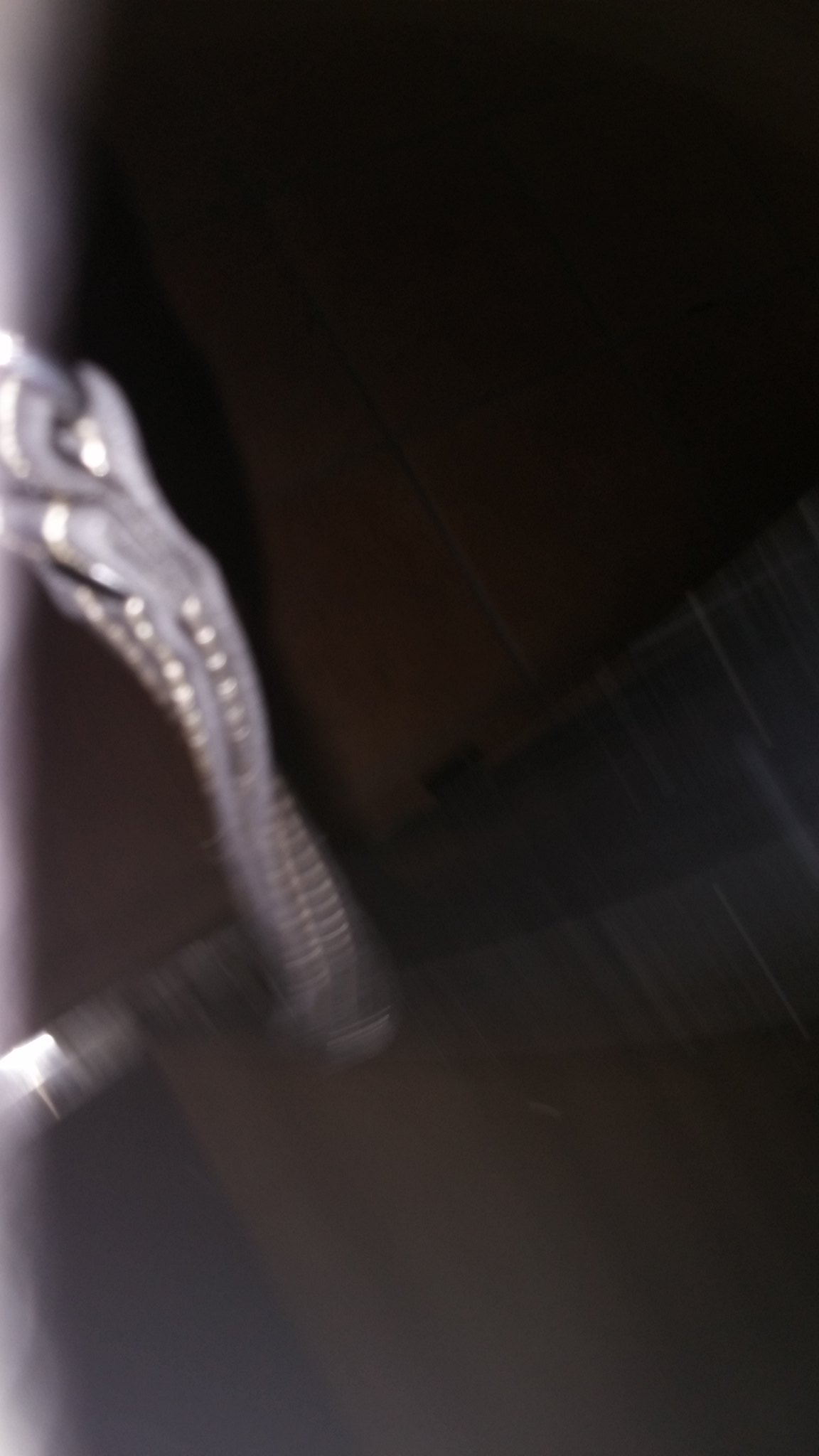The image features a predominantly blurry view with a complex mix of colors and shapes. The top portion is black, transitioning to a silvery, lighter gray with curved and textured strips in the middle. The image gives the impression of a twisted piece of metal running diagonally from the upper left portion and filling the center. Dark gray lines extend to the right, and the background shifts its hues: from brown at the top, changing to blue in the middle, and then back to brown at the bottom, which could depict a long brown door with a sliver of light underneath. In the lower left corner near this door, a navy blue stripe appears, adjacent to the brown floor. Additionally, there is a decorative table leg in the foreground, about six inches long, boasting a blue surface adorned with two vertical rows of silver diamonds.